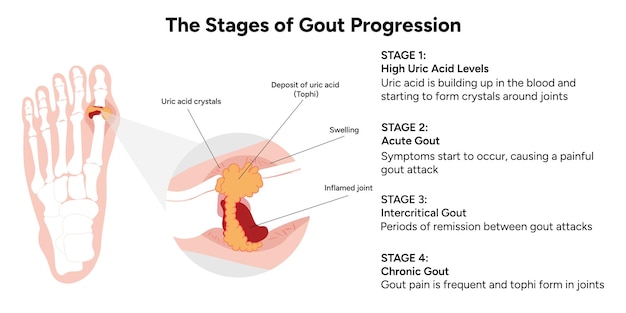The image is a detailed, color diagram illustrating the stages of gout progression. On the left side, it features a drawn x-ray of a left human foot, focusing on the joint just below the big toe. This area is shown in a magnified circular inset, highlighting various components like uric acid crystals and tophi, which appear as orange, bubbly clusters. Surrounding these deposits is maroon-colored inflammation closest to the bone and darker skin tissue indicating swelling. 

The right side of the diagram explains the four stages of gout: 
1. **Stage 1: High Uric Acid Levels** - Uric acid builds up in the blood, beginning to form crystals around the joints.
2. **Stage 2: Acute Gout** - Symptoms manifest, leading to painful gout attacks.
3. **Stage 3: Intercritical Gout** - Periods of remission occur between gout attacks.
4. **Stage 4: Chronic Gout** - Frequent gout pain with tophi forming in the joints.

Overall, the diagram effectively describes how uric acid buildup progresses through distinct stages of gout, causing considerable pain and joint damage.